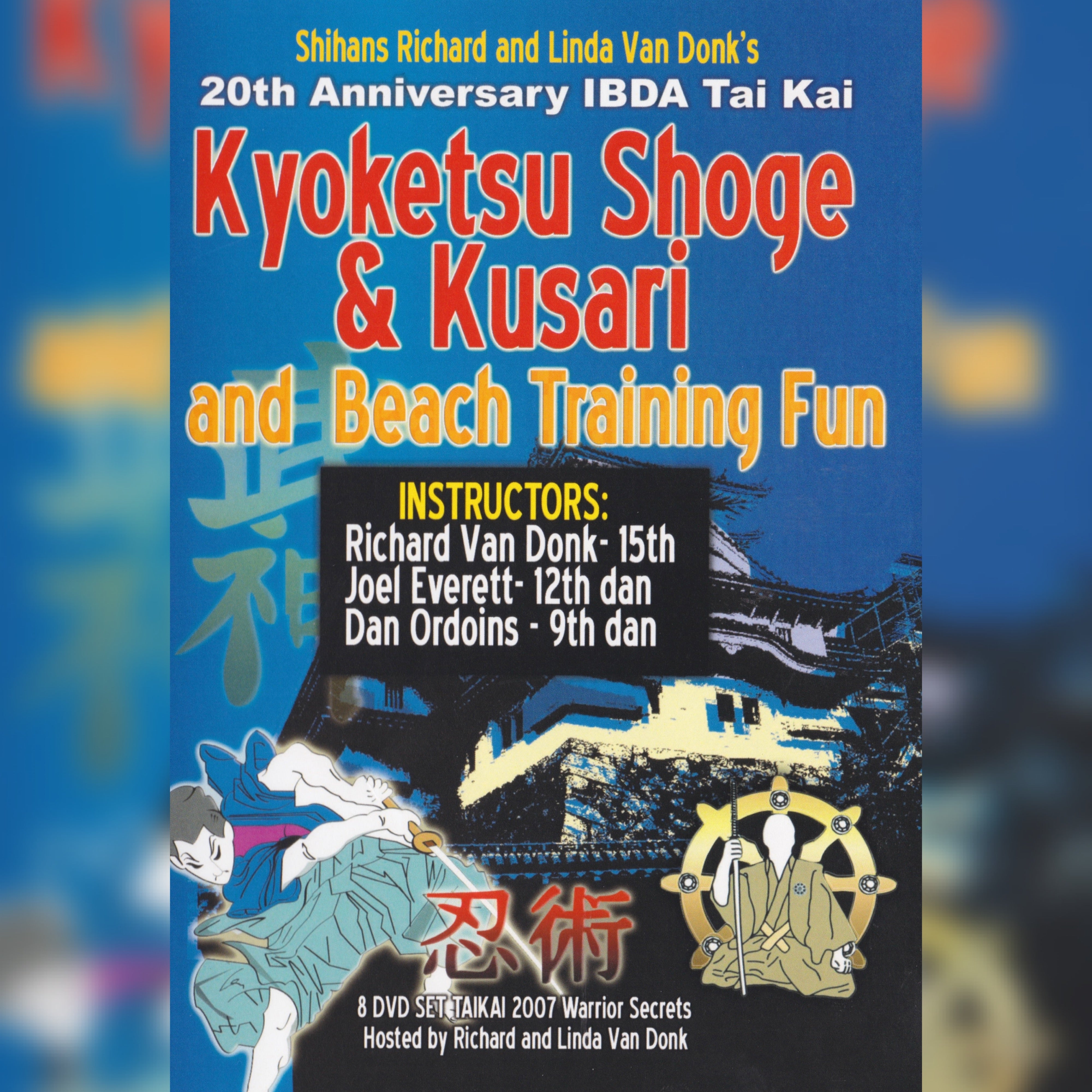The image is a blurred poster with a deep cobalt blue background and highlights in yellow and red, presenting an advertisement for a martial arts event. The focal point of the poster is a pagoda-topped building that appears silhouette-like in the mid-horizontal area. Above this, text reads "Shihan's Richard and Linda Van Donk's 20th Anniversary IBDA Taikai" in vibrant yellow and bold white print. Below this, large red lettering with a white outline announces "Kyoketsu Shoge & Kusari" followed by "End Beach Training Fun." At the bottom is a black horizontal rectangle featuring the word "Instructors" in yellow, with details of instructors beneath it: "Richard Van Donk - 15th Dan, Joel Everett - 12th Dan, Dan Ordoins - 9th Dan" in white text.

The visual elements include a cartoon graphic of an Asian male in the lower left corner, dressed in a dark blue top and light blue kimono-style pants, holding a gold-hilted sword. Nearby, there's Asian calligraphy in bold red with a white outline. On the right corner of the black bar is a gold ship's wheel with a sensei in a gold kimono sitting cross-legged in front of it. The bottom of the poster concludes with "8 DVD Set Taikai 2007 Warrior Secrets" in all caps, and "Hosted by Richard and Linda Van Donk" in bold white text.